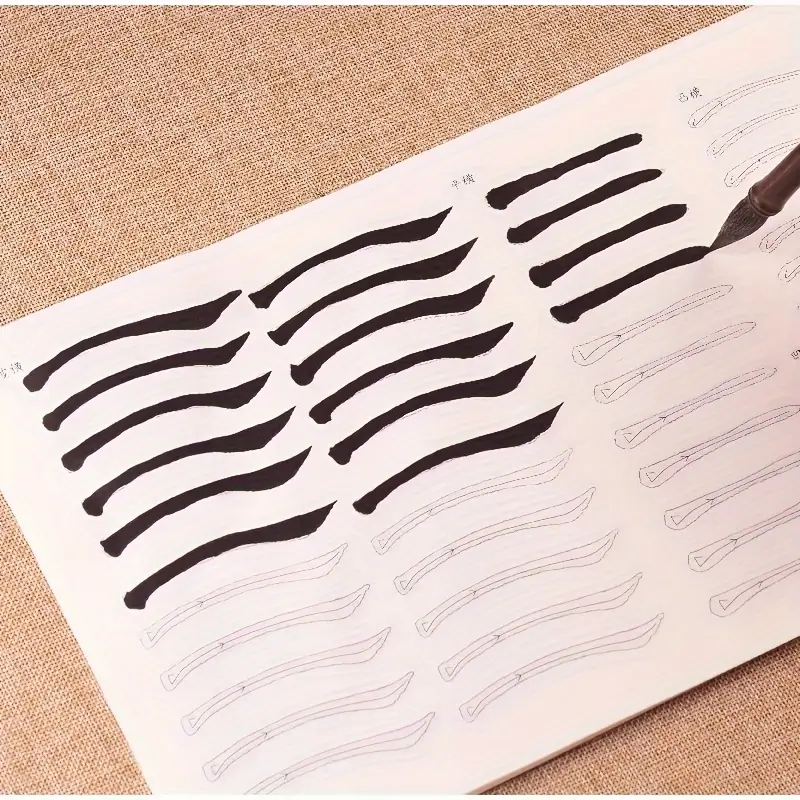This portrait-oriented photograph captures a meticulous moment of artistic practice. A booklet filled with outlines of various utensils – resembling small spoons or knives – serves as the focal point. Each utensil is being brought to life as an individual uses a calligraphy paintbrush to fill in the outlines with precision. Chinese characters are prominently displayed at the top of the booklet, hinting at a cultural or instructional context. The entire booklet is rendered in black and white, creating a striking contrast against the light brown, tan-colored fabric that it rests upon. The fabric appears textured, adding a layer of subtle warmth to the scene. There are four discernible rows of utensils, and curiously, the person filling them in seems to focus only on six items per row, leaving five more in each row untouched. This detail evokes a sense of process and progress in the meticulous study and application of traditional arts.